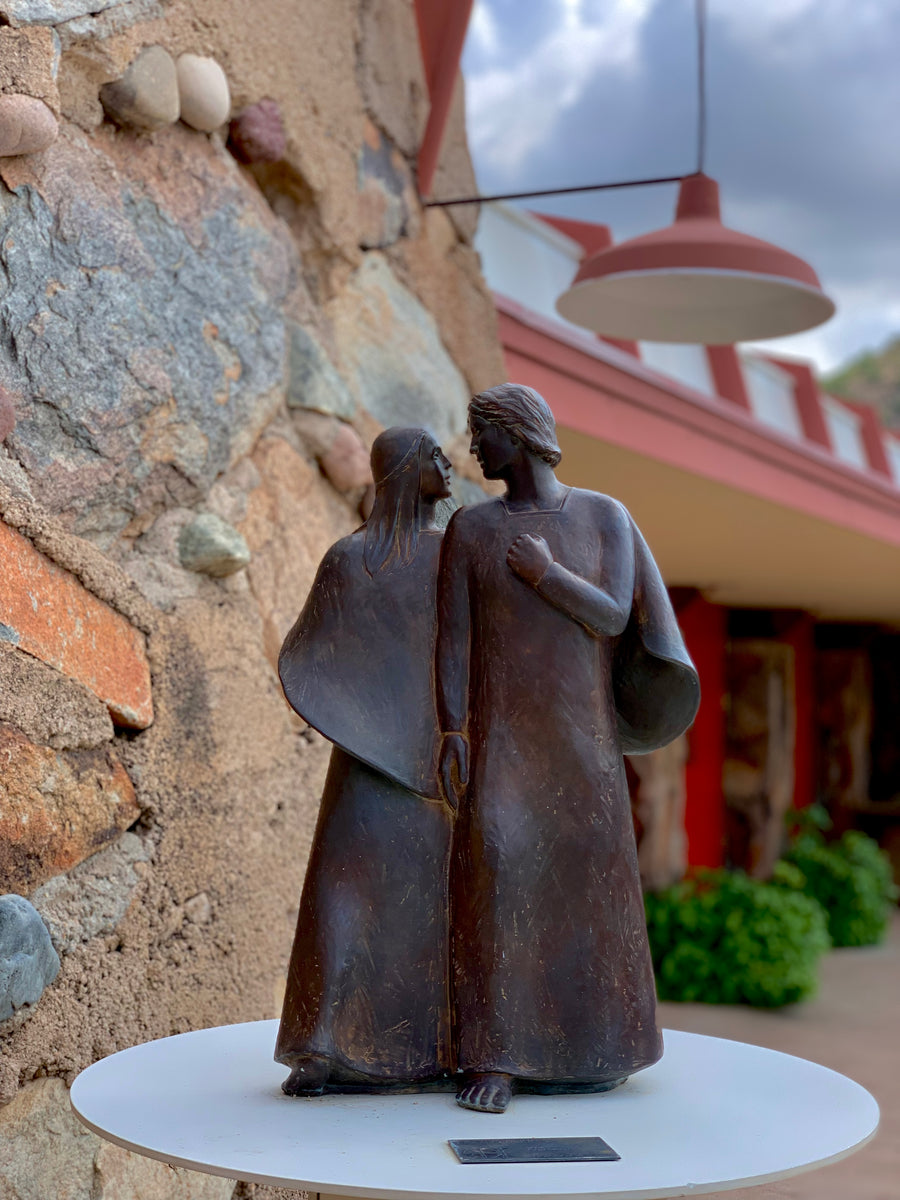The photograph, oriented in portrait mode, features a detailed metallic sculpture, likely made from patinaed bronze or iron, prominently displayed on a small, white, round table with a nameplate in front. The sculpture, approximately a foot tall, depicts a barefoot couple: on the left, a woman dressed in a shawl and long robe stands slightly behind a man on the right, who is similarly robed and caped. Her head is turned up towards him, while his body faces forward with his head turned back, his right arm resting against her chest and his left arm bent, fist over his heart. Both figures share a connected, intricate design. The backdrop includes a large stone building with a tan, blue, and melon-colored facade, featuring dark, cloud-filled skies above. The structure highlights its massive masonry and several red doors, accompanied by green shrubbery at the entrance.